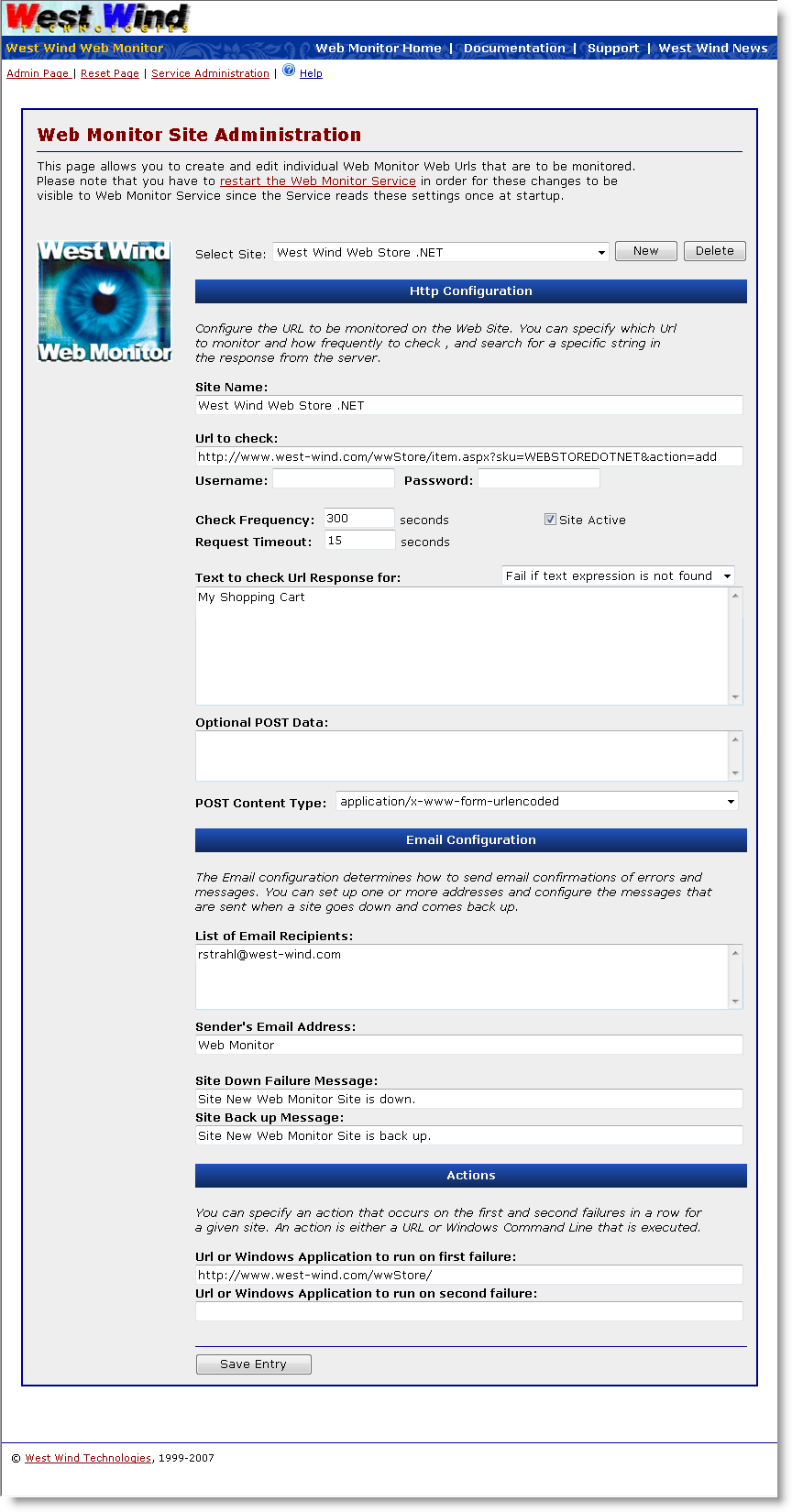This image is a detailed screenshot possibly taken from an online interface. The overall shape of the image mimics that of a cellphone screen, featuring a mostly white outer background transitioning to a gray middle section. A very thin line border surrounds the image, accented with subtle shadows to the right and lower right, giving it a slight pop-out effect.

In the upper left corner of the page, the stylized text "West Wind" stands out. "West" is written in red, while "Wind" is in blue, both capitalized and with angled black letters in between. To the right of this, a narrow, dark blue horizontal bar stretches across the width of the page. Within this bar, the words "West Wind Web Monitor" are inscribed in initial caps with an orange-yellow font. The right side of the bar features four white text sections separated by vertical lines: "Web Monitor Home," "Documentation," "Support," and "West Wind News," suggesting navigational links on a web page.

The main body of the image includes a larger white background area. Near the top left of this area, in the header, are three underlined orange-red links—"Admin Page," "Reset Page," and "Service Administration"—separated by vertical lines. To the right of these links, a blue question mark icon denotes a help section with the underlined blue word "Help."

Within the white section lies a gray background area bordered in blue, containing various interface elements. At the top left of this section, "Web Monitor Site Administration" is prominently displayed in burgundy text followed by a line running across the section's width. Under this header, left-aligned text explains the page's function, spanning three lines and including a clickable "Restart the Web Monitor Service" link in the middle.

On the left side below this header, a blue eyeball image icon is featured with "West Wind" written in white text at the top and "Web Monitor" at the bottom. The right half of the gray section is filled with a dense array of settings and fields. Toward the top center, a long white search bar labeled "West Wind Web Store.net" is flanked by "New" and "Delete" buttons on the right.

Three dark blue headers dominate the configuration area: "HTTP Configuration," "Email Configuration," and "Actions." Under each header, multiple fields and text sections appear. For the "HTTP Configuration," fields include site name input, URL checks, and other customizable settings. Under "Email Configuration," there are fields for email recipients and related settings. The "Actions" section contains fields for defining actions on first failure, with an associated HTTP address.

At the very bottom left, a button labeled "Save Entry" finalizes the image's plethora of menu items, input fields, and configuration options, representing a robust and complex web monitoring interface.